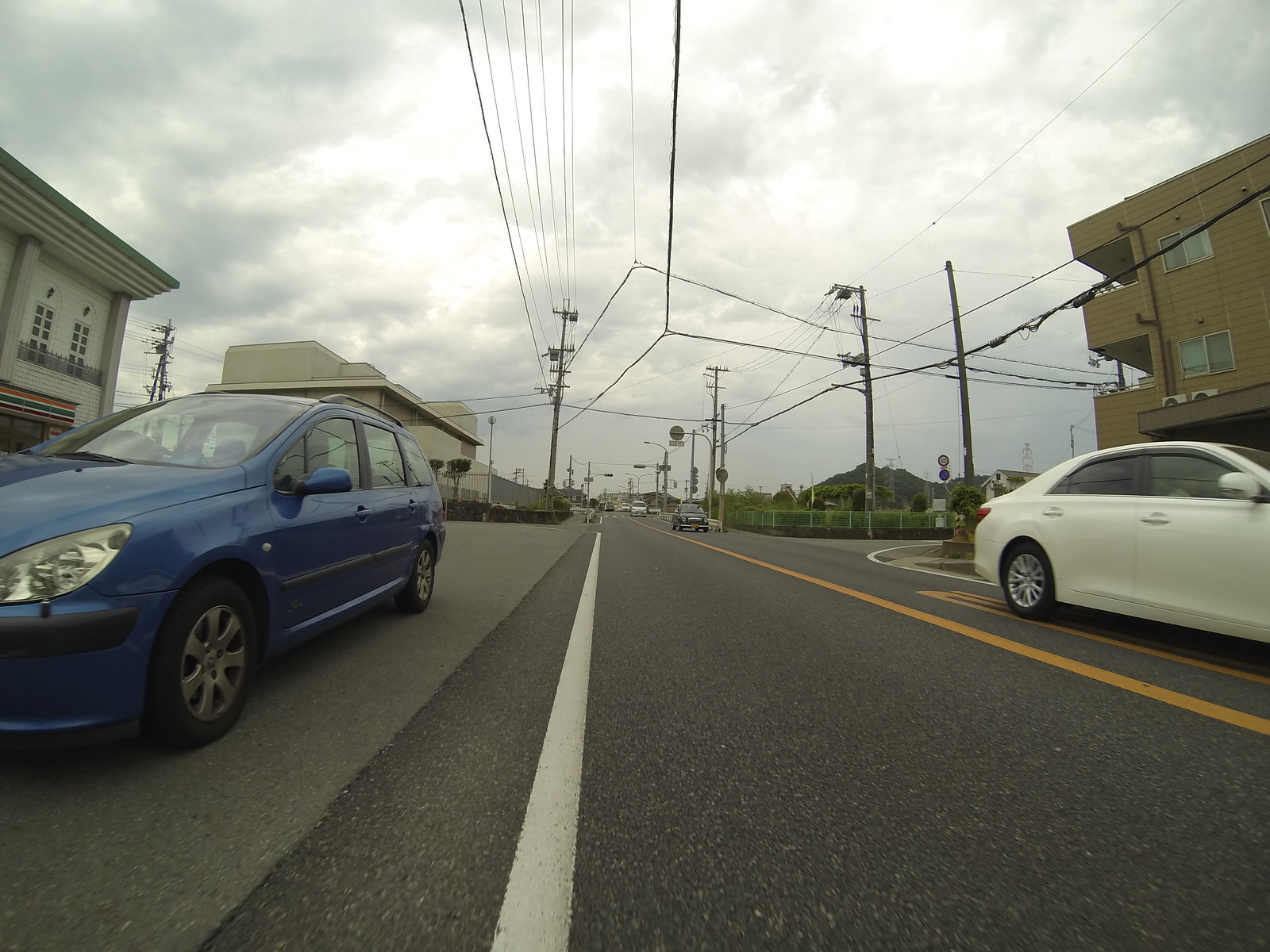This horizontally-oriented photograph, taken from the middle of a two-lane street in a residential neighborhood, captures a cloudy, overcast day. The gray, overcast sky looms above, setting a somber tone. On the left side of the road, there are two buildings and a blue car, facing towards the camera. Across the street, there is a white sedan positioned towards the bottom right of the image. The road, featuring a solid yellow line down its center, leads towards an intersection marked by power lines and timber posts on both sides, with additional cables crossing the junction. In the background, an apartment building stands prominently on the far side of the intersection, next to a green fence with another building behind it. The detailed composition highlights the everyday elements of urban life under a moody sky.